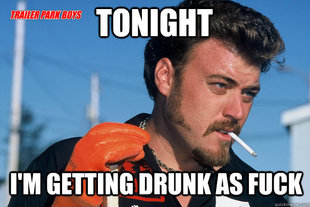This detailed image features an older, muscular, bald white man, possibly in his late 50s or early 60s, positioned on all fours in the center of a neatly made bed. He is shirtless, showcasing a tattoo on his right shoulder, and sports a salt-and-pepper beard that is closely shaved. The man wears only a black elastic belt with a small strap around his waist. Behind him, there are black pillows with white stripes. The bedspread is camo-print with a complex pattern of dark red, gray, black, and white, complemented by black sheets. The wall behind the bed is painted a very dark gray, and there is a light source reflecting off the wall, illuminating the scene. On either side of the bed, white electrical outlets are visible. In front of the man, a black pole with a white wing near the top protrudes below his tummy. A large text overlay in white capital letters spells "H.A.I." at the center front of the image.